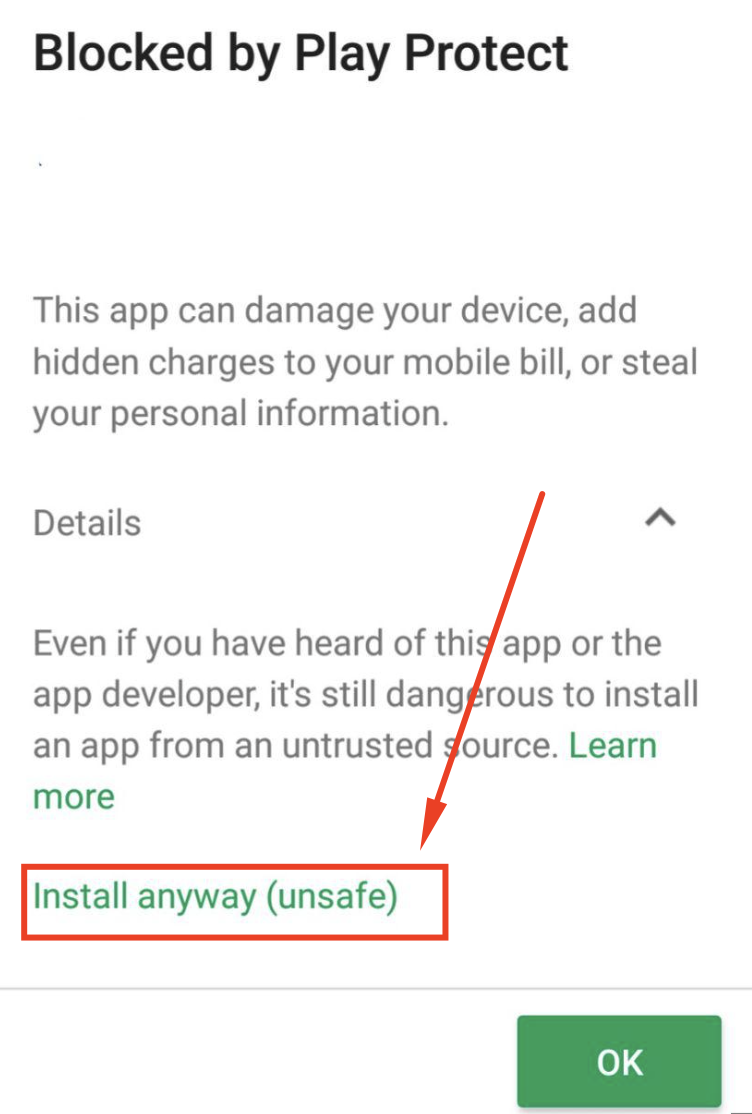This screenshot features a predominantly white background and contains a warning displayed by Google Play Protect. At the top, bold black letters spell out "Blocked by Play Protect." Approximately eight lines down, there is a gray three-line paragraph that reads: "This app can damage your device, add hidden charges to your mobile bill, or steal your personal information." 

About four lines below this message, in gray text, is the word "Details" accompanied by a black upward-pointing arrow (an upside-down 'V') on its right side. Four lines further down, another gray paragraph warns: "Even if you have heard of this app or the app developer, it's still dangerous to install an app from an untrusted source."

Below this warning, three lines down in green text, it says "Learn more." Another three lines down in green text is the option "Install anyway (unsafe)," which is outlined with a red rectangle. A red arrow, originating halfway up the screen and slightly left from the right edge, points downwards towards the "Install anyway (unsafe)" option.

Finally, at the bottom right corner of the screenshot, there is a green rectangle containing the word "OK" in capital white letters.